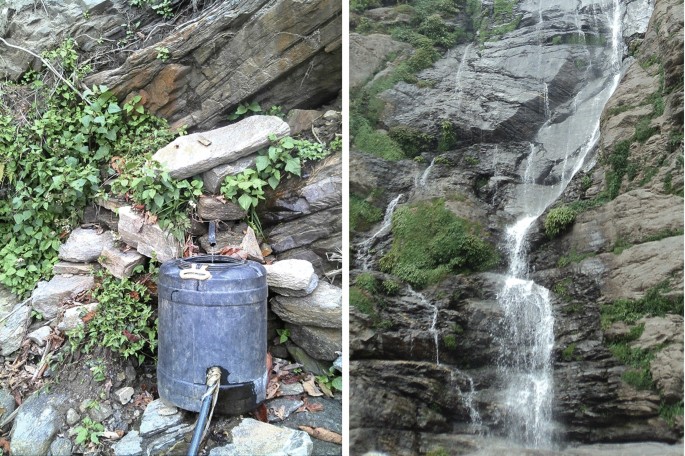The image is divided into two side-by-side photos, each depicting a different nature scene. The left photo features a rocky area with green leaves growing sporadically among the rocks. Some of the foliage appears vine-like, and there's a noticeable dense cluster of green in the middle-left section of the image. At the bottom-right of this scene sits a black bucket, which is connected to a hose leading out of frame. A black metal spigot juts out from an opening in the cliff, releasing a small stream of water into the bucket.

The right photo showcases a large, towering gray cliff with a narrow waterfall cascading from the top-right, flowing down towards the middle-bottom of the image. The cliff is covered in patches of green moss and sparse foliage, adding vibrant contrast to the gray rock. The waterfall itself is delicate, creating a picturesque stream amid the rugged, expansive rock face.